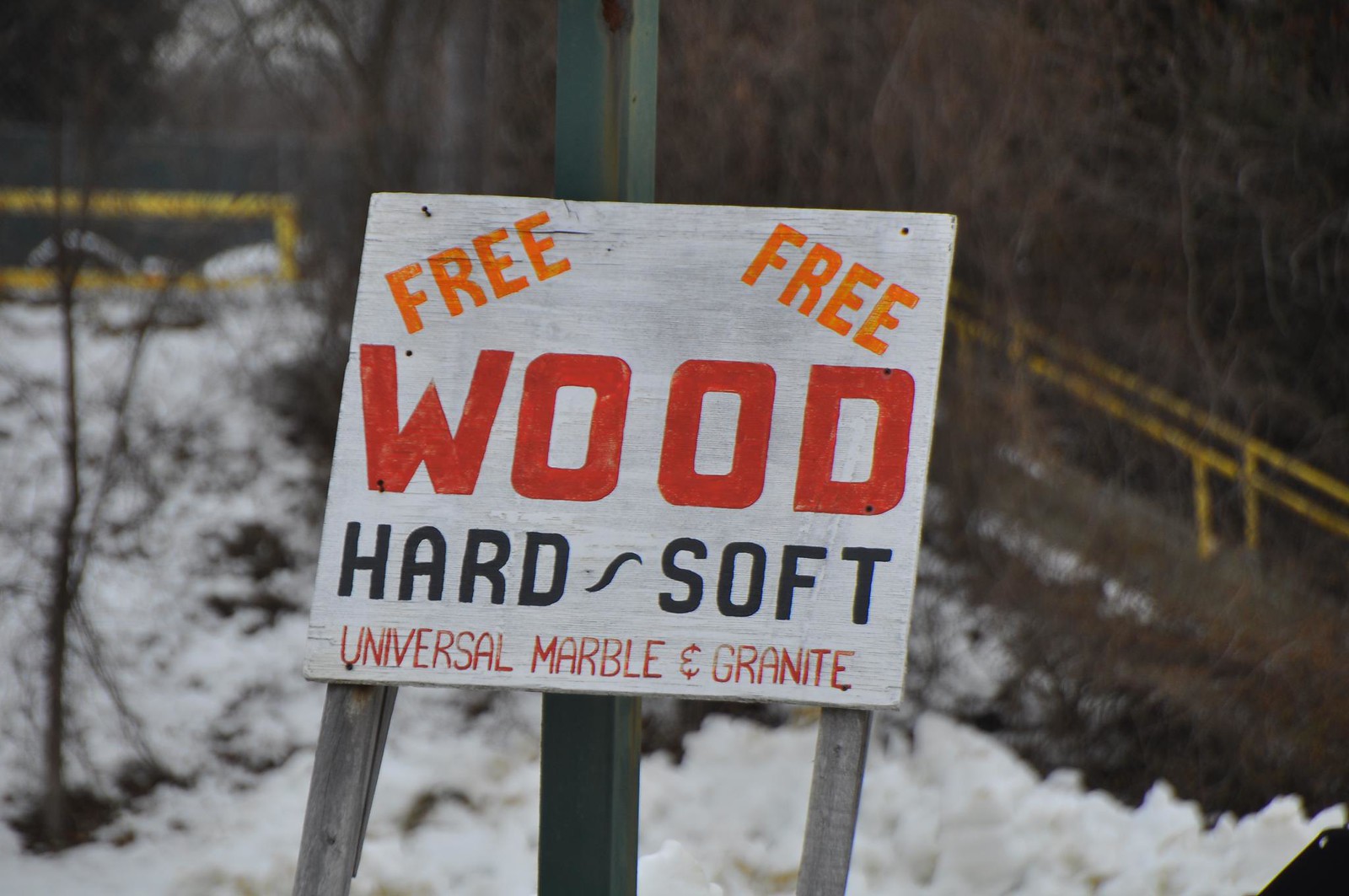This color photo, taken outside during the day, features a white wooden sign positioned against a green post in a snowy environment. The white sign prominently displays the words "Free," "Free," "Wood," "Hard," "Soft," "Universal Marble and Granite" in various colors: "Free" is angled and written in orange on both sides, "Wood" in bold red, "Hard" and "Soft" in black, and "Universal Marble and Granite" in a lighter red. The sign, no longer fixed but rather leaned against the post, has metal or wooden poles suggesting it was once firmly planted. In the background, there are bare trees, dried-out plants, snow-covered ground, and a distinctive yellow railing that encloses a walkway and staircase. The scene suggests a connection to forestry, possibly indicating a source of the advertised materials.